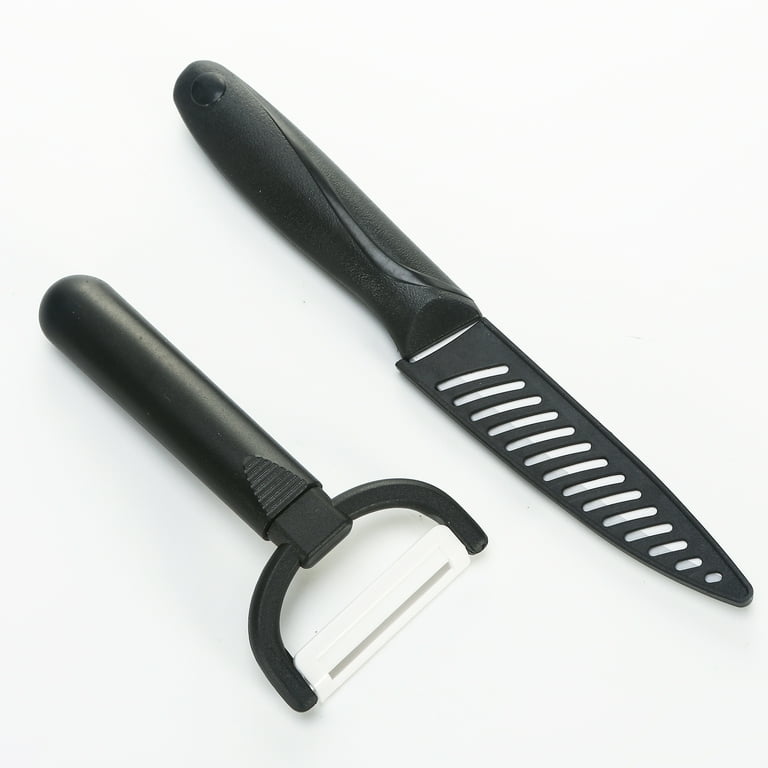In the image, set against an almost white, very light gray background, two kitchen utensils are positioned diagonally with their handles in the upper left and their functional ends pointing towards the lower right. The upper utensil is a knife with a sturdy black plastic handle that has a textured grip. The knife blade is sheathed in a black cover adorned with diagonal slats, allowing glimpses of the silver blade beneath. Below the knife is a potato peeler with a black plastic handle leading to a white blade, affixed to a curved black piece. The meticulous arrangement and the high-quality appearance of these utensils suggest they might be part of an advertisement.